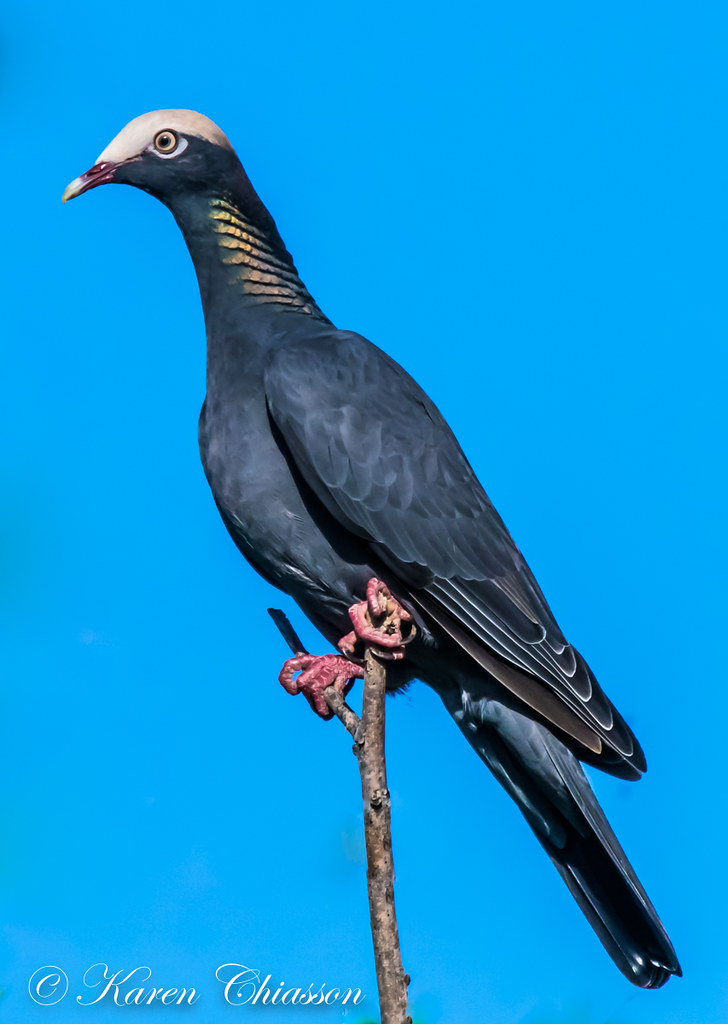This is an image of a bird, specifically a dark gray bird with a striking appearance, captured outdoors during the day by Karen Chiasson, as indicated by the copyright notice in the lower left corner. The bird is perched on a bare Y-shaped branch against an aqua blue sky. The bird's head is adorned with a white band that stretches from the top down to just above its eye, which is encircled by a white ring. The bird has a long, stretched-out neck that prominently features several lines of almost reflective, yellow feathers, creating a series of gold striations. 

The bird's beak is dark brown with a yellow tip, and its eyes are yellow. Its body is primarily dark gray with white-tipped wing feathers, and the bird has a very long tail. The red legs and pink claws grasp the branch firmly, creating a poised profile. This bird has a blend of silver, gray, and green highlights on its neck, adding to its unique and beautiful appearance.